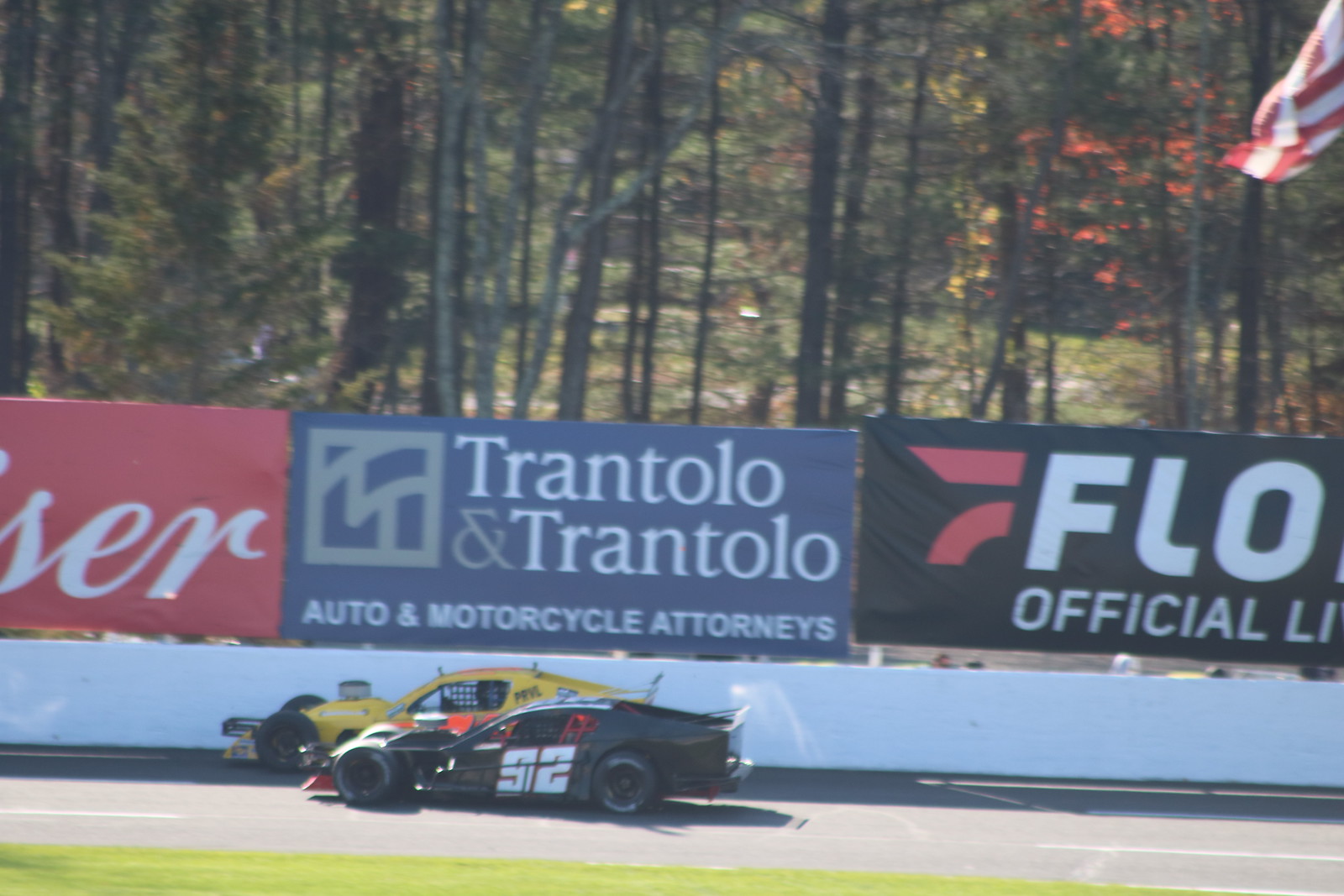The image captures an intense moment on a race track during daytime, featuring two race cars in motion. Closest to the viewer on the track's lower left-hand side is a sleek black car marked with the number 92 in white. Slightly ahead of it, on its right, is a bright yellow car. The cars are racing on the dark asphalt track, bordered by a short white wall that extends horizontally across the image. Beyond this wall, large billboard advertisements are visible; the one on the left, partially cut off, has "S-E-R" in white letters on a red background, likely indicating Budweiser. The central billboard is blue with "Trantolo and Trantolo" in prominent white letters, followed by "Auto and Motorcycle Attorneys." To the right, a black billboard features the letters "F-L-O," and below that, "Official L-I" can be vaguely seen. The background includes a dense forest area with trees displaying autumn foliage in green, yellow, and red hues. A glimpse of an American flag's red and white stripes is visible in the top right corner of the image. The track's infield shows patches of grass and exposed brown dirt, setting the scene as an exciting and vibrant motorsport event.